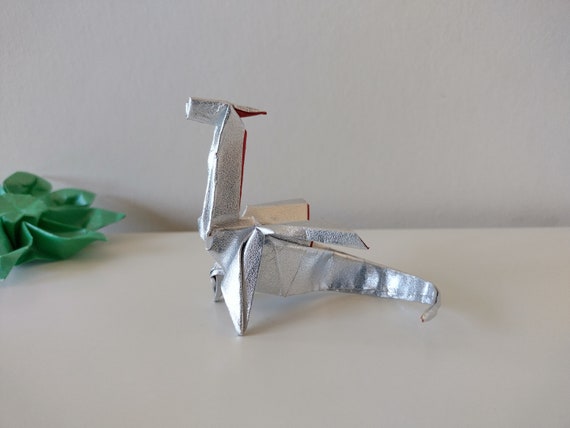In the image, a meticulously crafted origami dragon, fashioned from silver or tinfoil paper, sits proudly on a white countertop against a light gray wall. The dragon features a long neck, a sharp, rectangular head with an ear jutting out behind, a triangular body, and intricately folded wings that twist and extend from either side. To the left of this central figure is another origami creation, a lotus flower made from green paper, with a solid center surrounded by delicately folded petals. The scene is elegantly composed, highlighting the contrast between the shiny, textured surface of the dragon and the smooth, vibrant green of the lotus flower.